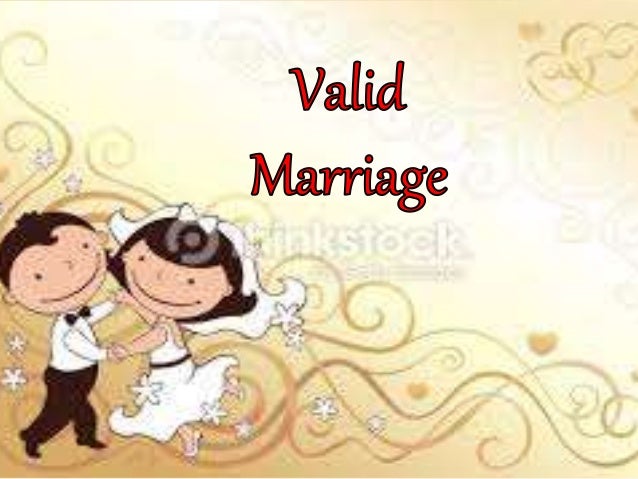This image is a vibrant cartoon drawing depicting a joyful married couple, prominently featuring the words "valid marriage" printed in red at the top center. The background is an alternating pattern of yellow and white. In the bottom left corner, the bride and groom are captured in a whimsical style, both with exaggerated, wide smiles. The groom is dressed in a white shirt, black bow tie, and black pants. The bride wears a white wedding dress, adorned with a veil and a white butterfly bow on top of her hair, and a belt around her waist that complements the groom's bow tie. Surrounding the couple are decorative elements, including curvy lines, swirls, asterisks, and stars, with hearts positioned at the top right. The overall design exudes a cheerful and celebratory vibe, suggesting that the image might be used for a congratulatory wedding card.